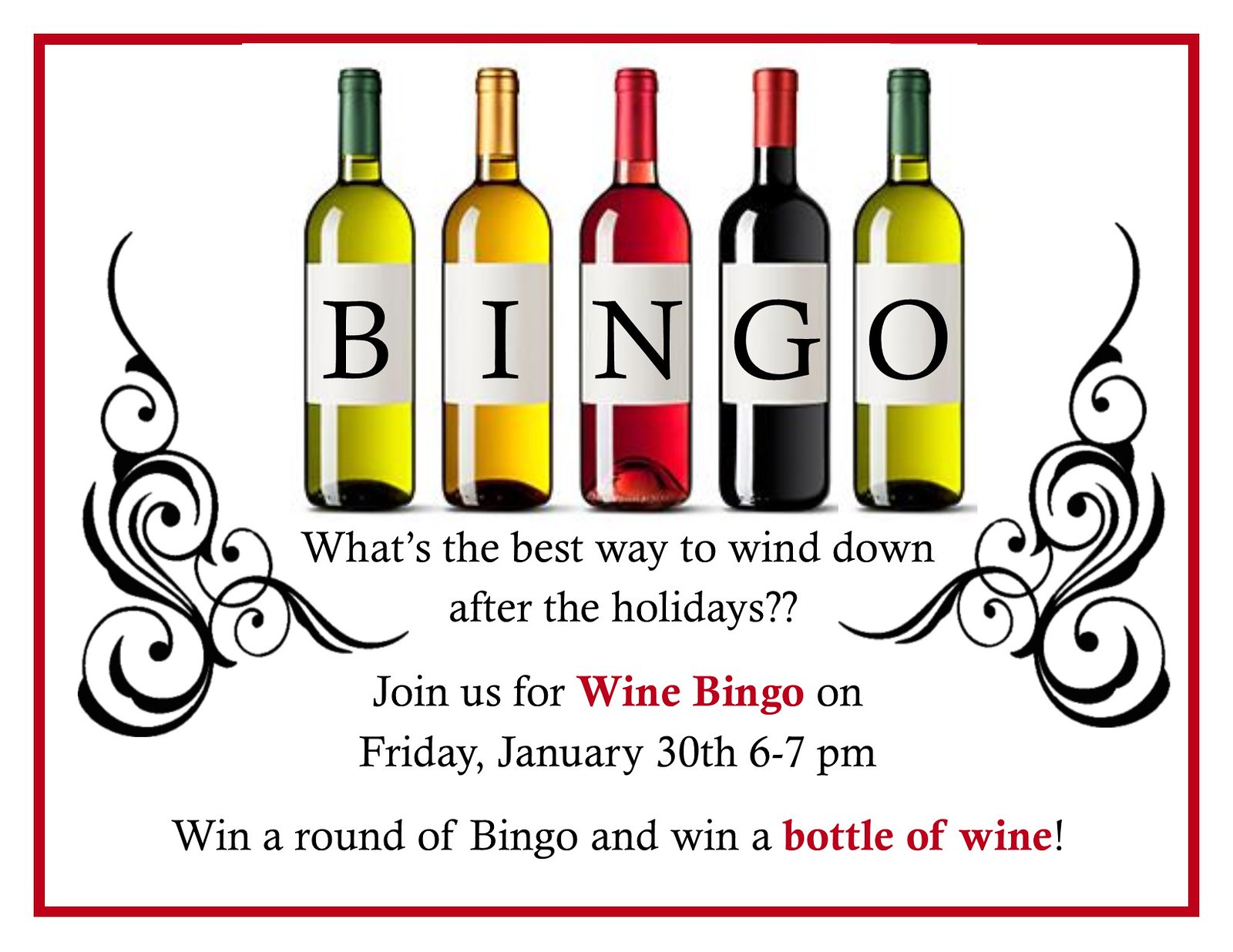This is a vibrant advertisement for a Wine Bingo event featuring a clean white background with a striking red border. Prominently displayed at the top of the ad are five artistically rendered wine bottles, each uniquely colored and topped, aligned to spell out "B-I-N-G-O." The leftmost and rightmost bottles share an olive green hue with dark green lids, while middle bottles include a gold-hued bottle with a gold lid for the letter "I," a cherry red bottle with a red lid for "N," and a rich black bottle with a red lid for "G." 

Interspersed with playful squiggly lines and curlicues, the text invites readers with the question: "What's the best way to wind down after the holidays?" In bold black font, it announces, "Join us for Wine Bingo," with the words "Wine Bingo" strikingly highlighted in red. The event details follow: "Friday, January 30th, 6 to 7 p.m." The call-to-action is clear: "Win a round of bingo and win a bottle of wine," with "bottle of wine" also emphasized in red, adding to the visual appeal and allure of the offer.